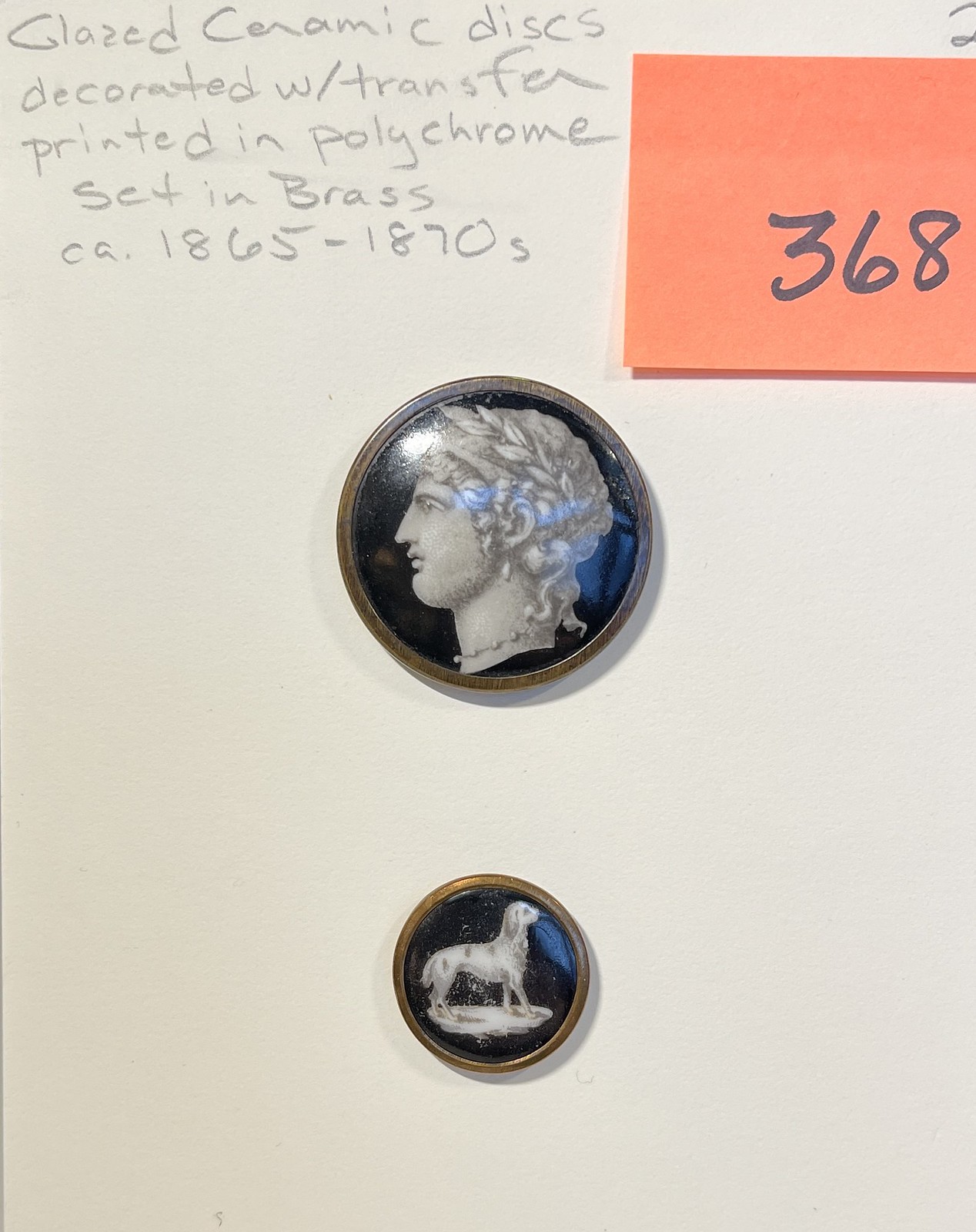This image features a light cream-colored sheet of paper showcasing two collectible items that appear to be Roman or Greek in origin. The paper has a detailed pencil inscription on the upper left that reads, "Glazed Ceramic Discs Decorated with Transfer Printed in Polychrome Set in Brass, CA 1865-1870s." On the upper right corner, there’s an orange post-it note with the number 368 written in black marker, alongside a small number 2 in pencil. Centered on the paper are two circular brass-outlined objects. The first object displays a side profile of a person's face with curly hair styled in an updo, against a black background. The head is rendered in a whitish color. Below, there is a second circular item with a small white silhouette of a dog standing on a white platform, also set against a black background. The dog features a few gray dots on its side.